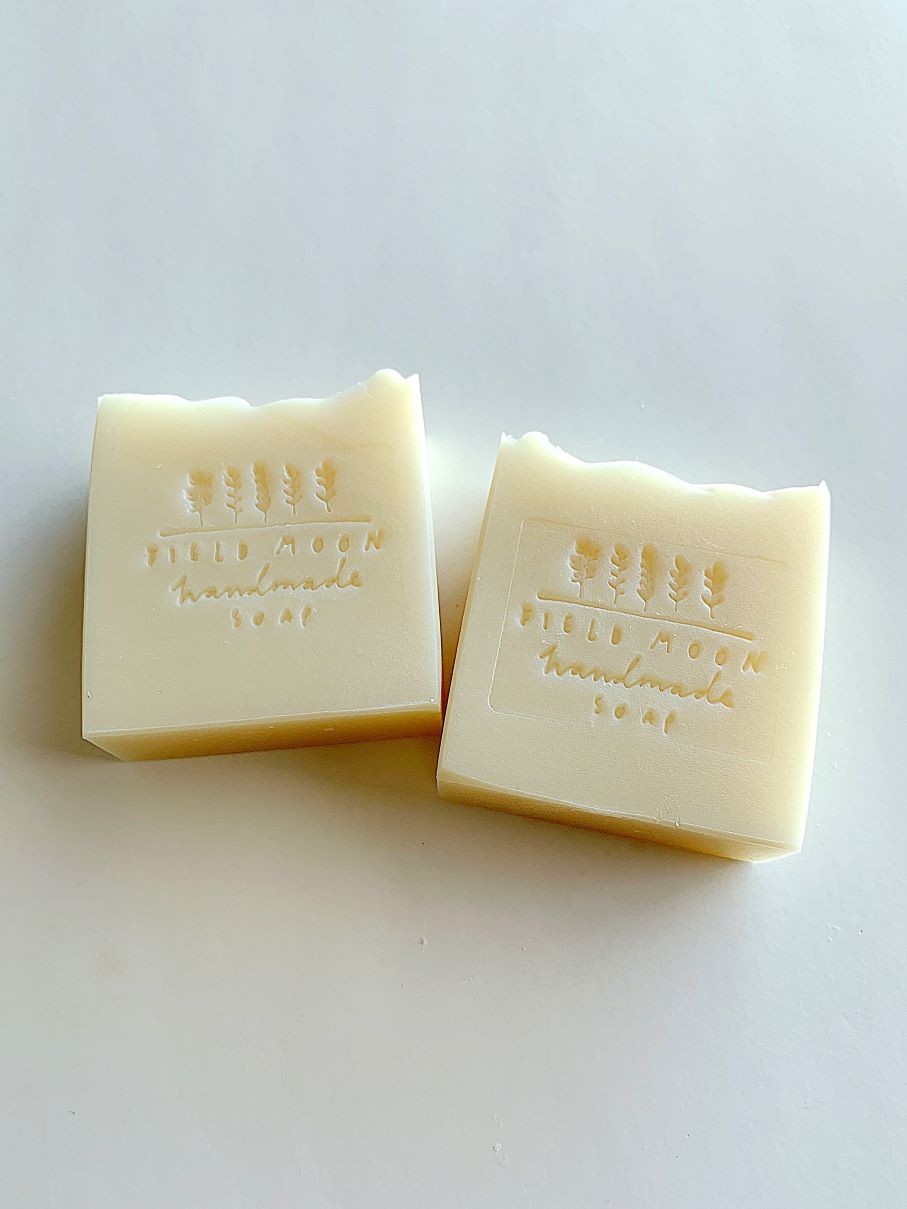This image is a detailed product photograph showcasing two handmade artisanal soap bars. The soaps are a creamy beige color and are set against a solid white surface, possibly a tabletop or a paper background. Both bars are rectangular in shape with three smooth, squared-off edges, while the top edge is jagged and uneven, likely intentionally left that way to give a natural, handcrafted appearance.

Etched into each soap bar is a detailed design featuring five leaf-like motifs arranged above a horizontal line, followed by the text "FIELD MOON" in a bold uppercase font. Below this, in cursive script, it says "handmade," and underneath that, in uppercase letters again, it reads "SOAP." The bar on the right has this logo within a more structured border, whereas the bar on the left does not. Both bars are identical in size, design, and color, although they might give the impression of being two halves of a previously whole bar due to their matching irregular top edges. Overall, the soaps exude a rustic, handcrafted charm.